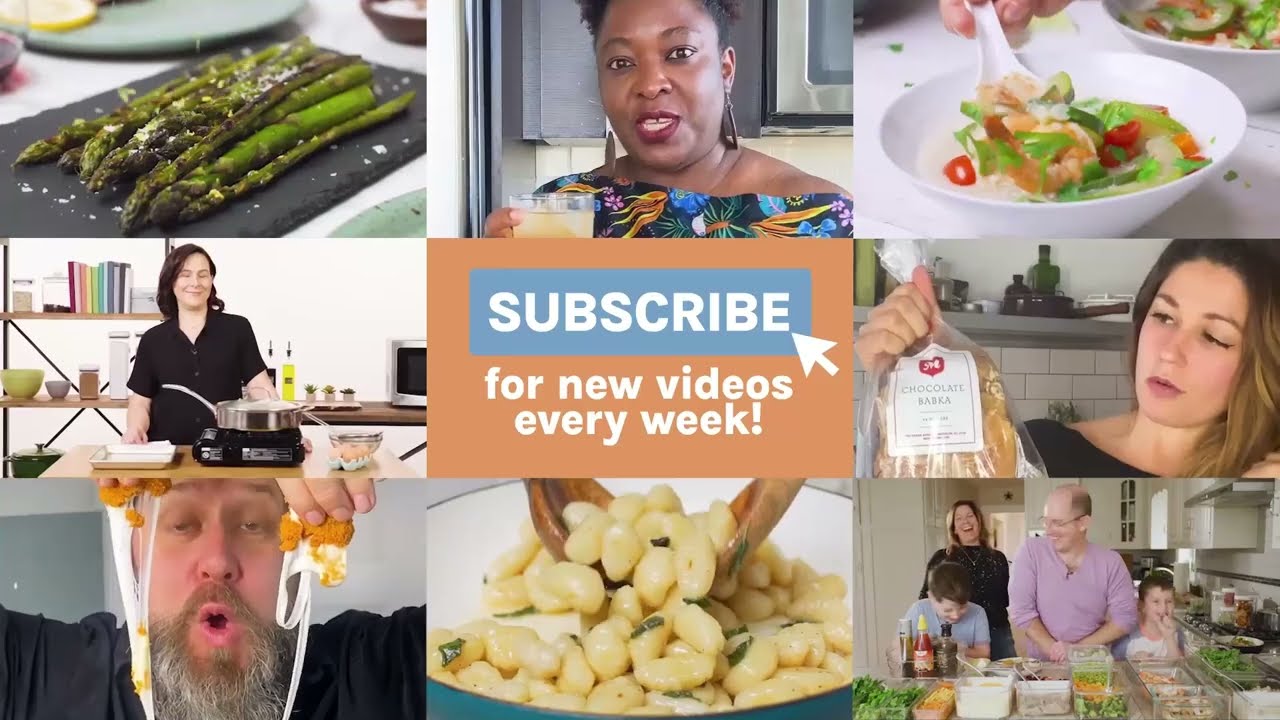The image is a 3x3 grid of rectangular photographs, each depicting a food-related scene, with an emphasized central block featuring an orangish-brown background and a blue rectangle labeled "Subscribe." Below the subscribe button, text reads "for new videos every week." The top left image shows a close-up shot of cooked asparagus with shredded cheese. The top middle block captures an African American woman holding a glass of lemonade and speaking directly to the camera. The top right photo presents a white bowl filled with salad, with a hand holding a white spoon above it. Moving to the middle row, the left block depicts a Caucasian woman with shoulder-length brown hair, wearing a black short-sleeved button-up T-shirt, standing behind a countertop with various cooking items. The center block prominently displays the subscribe button along with the accompanying text. The middle right image shows another Caucasian woman with dark brown hair streaked with lighter tones, holding a bag of bread. The bottom left image features a Caucasian man with a large white and gold beard, holding a fried, cheese-filled treat with melted cheese stretching out. The bottom middle photo highlights a pan with cooked garbanzo beans, tossed with herbs. Finally, the bottom right image captures a joyful family of four - a man, a woman, and two kids - crowded around a kitchen counter and engaging in a cheerful meal.